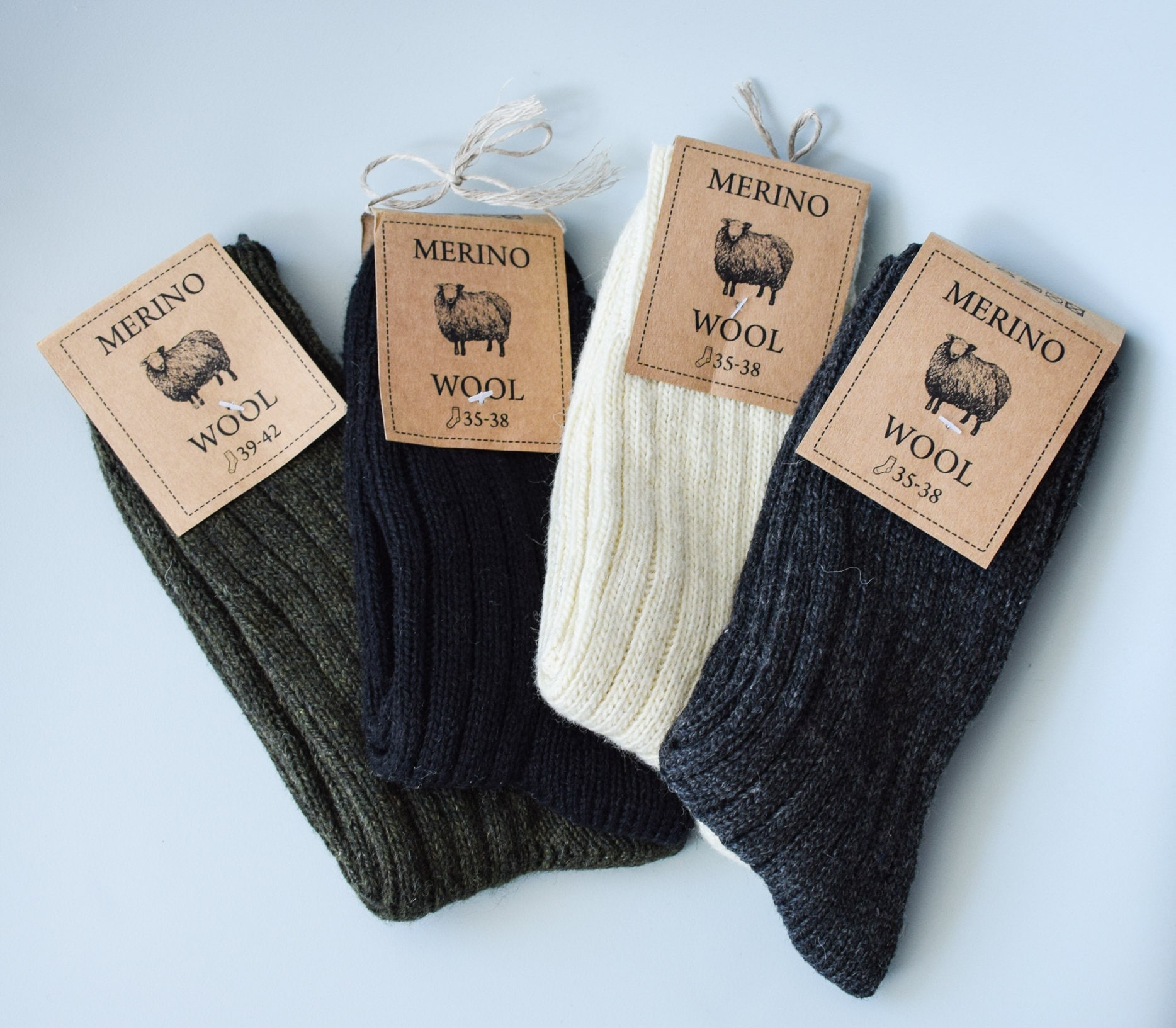The image features four pairs of merino wool socks neatly arranged side by side against a light blue background. Each pair of socks is attached to a beige label with black print, reading "Merino Wool" at the top, accompanied by a silhouette of a sheep. Below the sheep image, the label displays the sock sizes.

The pair on the far left is dark gray and labeled size 39 to 42. Moving right, the next two pairs are navy blue and off-white, both labeled size 35 to 38, and adorned with thread bows. The pair on the far right is a blue-gray mix, also size 35 to 38. Each label is secured to the socks with a small poking device or string, ensuring the tags stay in place. The consistent branding and concise size information make the socks easy to compare and identify.